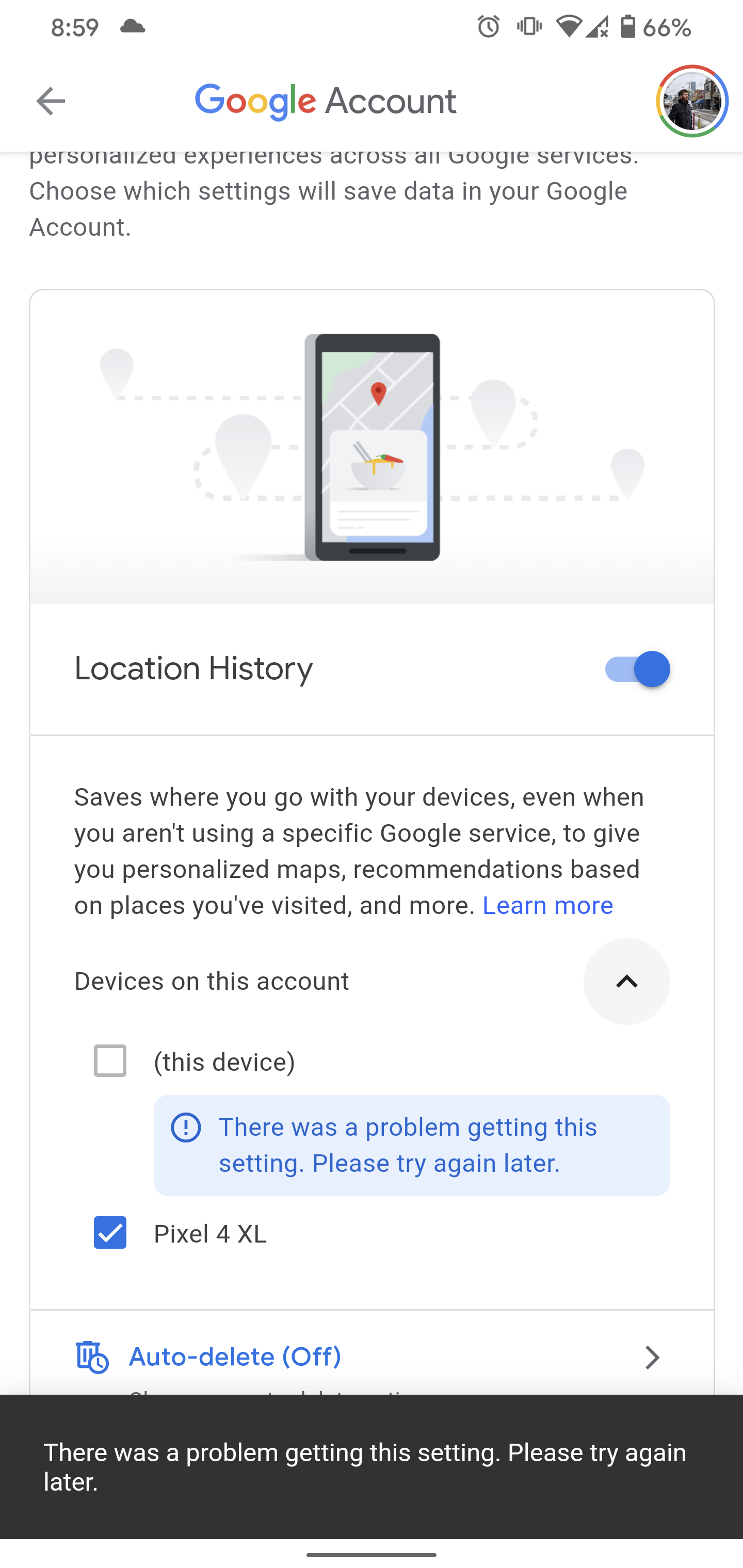The image is a vertical screenshot from a cell phone display, with dimensions approximately three times taller than it is wide, predominantly featuring a white background. In the upper left corner, the time "8:59" is displayed in black text, accompanied by a cloud icon. On the upper right side, several status icons are visible: an alarm icon, a vibrate icon, cellular coverage showing about three-quarters strength, and a wireless coverage icon marked with an 'X' indicating issues. The battery icon shows a charge of roughly two-thirds, indicating "66%".

Moving down, on the left-hand side, there is a back arrow, followed by the word "Google" in the company's signature multicolored logo style. Next, the word "Account" is written in black, situated to the right of the Google logo. Adjacent to this is a profile picture, implying user login information.

The content below suggests the user has scrolled down as the screen captures part of an ongoing paragraph, leading into a new section that is highlighted with a gray rectangular border. This section features an image of a cellphone displaying a bowl of ramen, with a Google Map above it showing a pin drop, indicating a search for a ramen shop. Beneath this image, the text "Location history" is present along with a toggle switch set to "on". A paragraph of text underneath explains this feature in further detail.